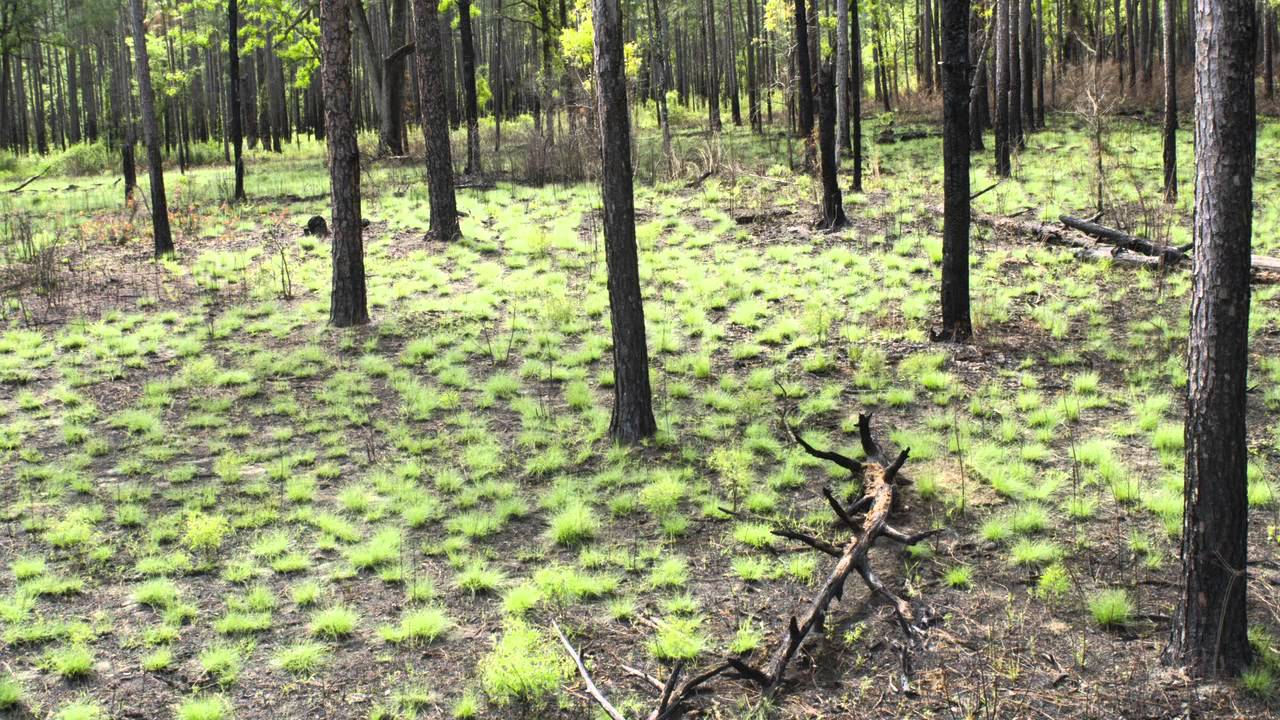The image is a color photograph in landscape orientation, capturing a forest scene with a mix of recent fire damage and natural regrowth. The forest floor is a patchwork of dark, rocky soil interspersed with clusters of bright green, mossy grass, hinting at new growth emerging after what seems to have been a recent fire. Numerous slender pine tree trunks dominate the foreground, extending from the ground up to about halfway, with their bark appearing dark gray to black, indicative of fire damage. The bottom portions of these trees are particularly charred, while some have grayish hues and lack branches or leaves, likely burned off by the fire. Scattered around are fallen tree limbs and branches, many of which are broken and stripped of foliage, particularly noticeable is a large curved branch in the bottom right, presenting jagged protrusions from where smaller branches were either broken or cut off. Towards the upper right section of the photograph, there are smaller, regenerating trees. The background becomes dense with more trees, their trunks blending into a mass of grayish-brown colors, and a few in the distance show vibrant leaves, offering a contrast to the stark barren foreground. The image portrays a realistic, detailed snapshot of a forest resiliently bouncing back from the aftermath of a fire.